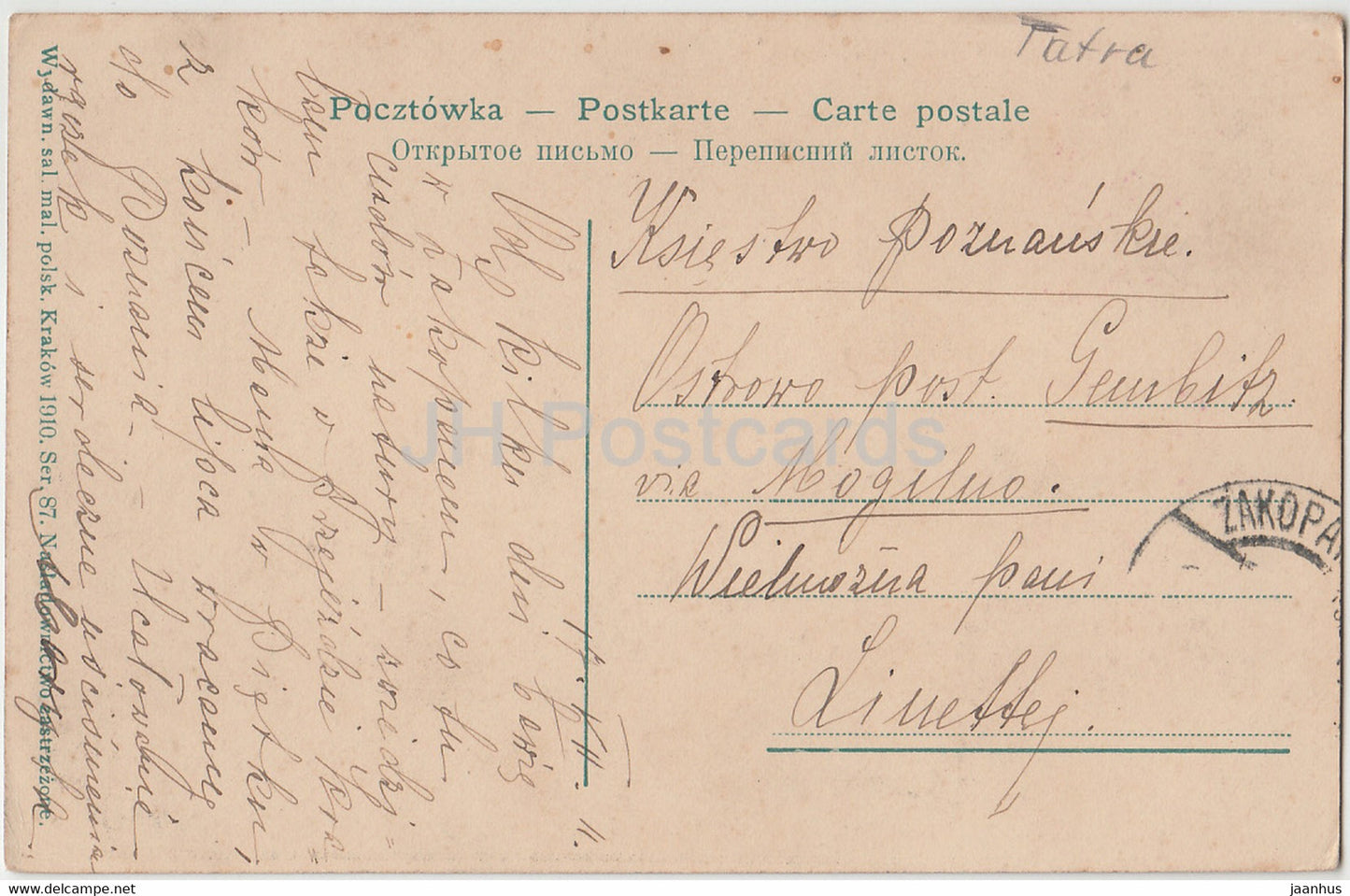The image showcases a beautifully detailed postcard, featuring an elegant handwritten message in an updated cursive font. The handwriting is sophisticated and fancy, adding a touch of personalization to the postcard. The rectangular shape of the postcard is clearly visible, enhancing its classic, nostalgic appeal.